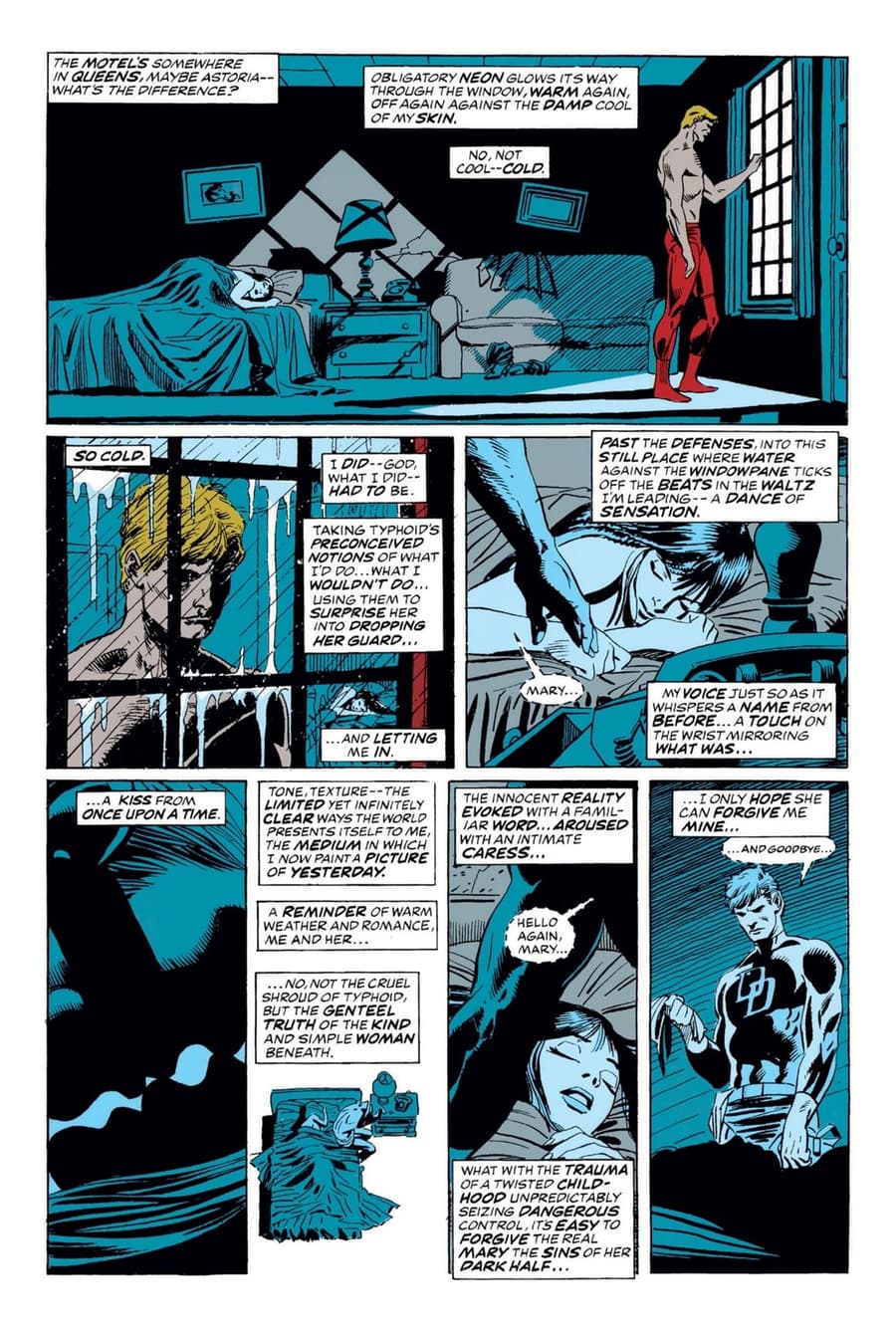This is a detailed comic book page comprising six panels, dominated by a monochromatic blue and gray palette with sporadic splashes of red. The large top frame features a pensive scene in a dimly lit bedroom where a man with yellow hair, dressed in red pants, stands at a window, peering out into a rainy night. His contemplative stance is accentuated by a series of narrative boxes with white backgrounds and black text, which provide a rich, introspective monologue. A woman lies in the bed behind him, her face often highlighted in the subsequent panels.

Moving through the frames, we see varying close-ups of both characters, capturing the man's troubled expressions and moments where he gazes back at the woman, causing a palpable emotional tension. The middle panels continue to toy with perspective, including an overhead view of the bed, laden with more narrative boxes that delve into his thoughts.

The final frame depicts the man in a superhero costume, emblazoned with the letters "DD," clearly identifying him as Daredevil. This transformation marks a poignant farewell moment as he gently interacts with the woman, tenderly kissing her and seemingly preparing to leave for another perilous night of crime-fighting. The powerful text, combined with the visual elements, captures a narrative oscillating between personal regret and relentless duty, set against the atmospheric backdrop of a neon-lit cityscape.